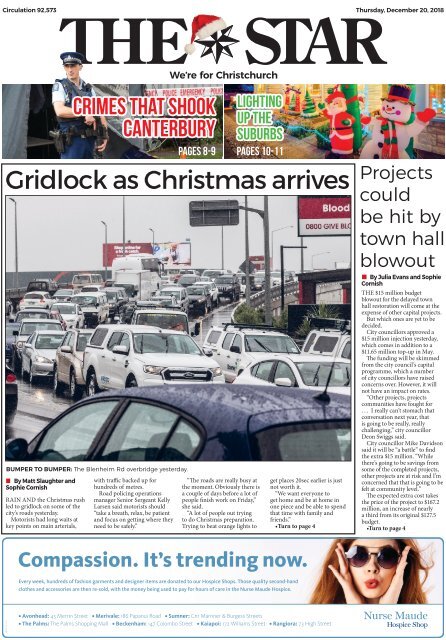This is a screenshot of a website designed to resemble a traditional newspaper. The background is predominantly white. In the upper left corner, the circulation is listed as "92,575." The upper right corner displays the date, "Thursday, December 20th, 2018."

Prominently featured is the newspaper's title, "The Star," written in very large font. Between the words "The" and "Star" is a unique graphic of a seven-pointed star adorned with a Santa hat. Below the title is the slogan, "We're for Christchurch."

Below this, there are two photos side by side. The photo on the left features a white male policeman dressed in an English police uniform, suggesting a setting in England. The accompanying text reads, "Crimes that Shook Canterbury," with a note to see pages 8 and 9 for more details. The photo on the right showcases festive Christmas decorations, specifically large inflatable yard ornaments such as Frosty the Snowman and Santa Claus placed in front of a house. The caption states, "Lighting Up the Suburbs," directing readers to pages 10 and 11 for the full story.

The top headline of the page is "Gridlock as Christmas Arrives," accompanied by an image depicting heavy traffic congestion.